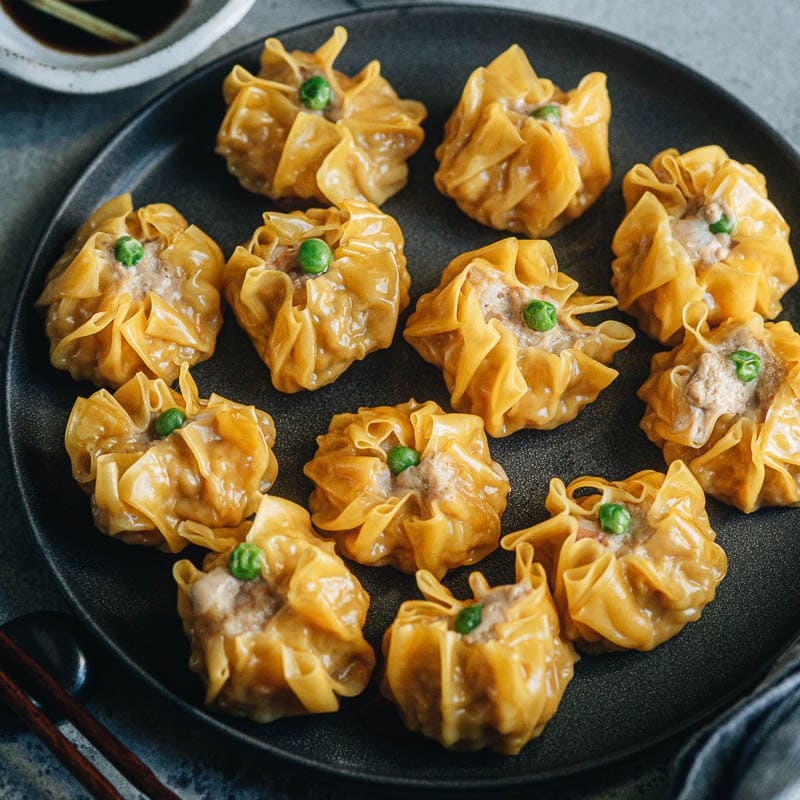This close-up, overhead angled shot captures a visually appealing arrangement of 12 wontons on a circular black stone plate. The plate rests on a stone gray table and each wonton features a browned, crispy skin, hinting at baking. The wontons are stuffed with a smooth, tan-colored filling that is possibly crab or tuna-based. A single green pea is meticulously placed at the center of each wonton, adding a pop of color. In the upper left corner of the frame, there is a white stone bowl containing soy sauce. Brown wooden chopsticks are seen laid diagonally on a black chopstick rest in the bottom left corner, while in the bottom right corner, blue and black cloth napkins add to the composition. The overall presentation is elegant and well-balanced, highlighting the artistry of the dish.